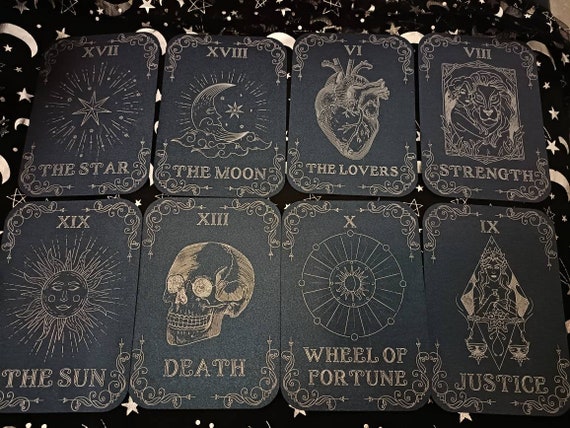This photograph showcases eight tarot cards arranged evenly in two rows of four against a black background, which features a faint, blurry astronomical or astrology pattern. Each card is black with silver or gray pencil sketch-like illustrations and Roman numeral labels. Starting from the top left, the first card is XVII, "The Star," depicting a radiant star in the center. Next is XVIII, "The Moon," showcasing a smiling moon. The third card, VI, "The Lovers," features a realistic human heart, not a typical heart symbol. The fourth card is VIII, "Strength," illustrating a woman holding a lion. The bottom row begins with XIX, "The Sun," showing a sun with rosy cheeks. Following this is XIII, "Death," marked by a skull image. Then, X, "The Wheel of Fortune," represented by a wheel. Finally, IX, "Justice," shows Lady Justice balancing scales. The detailed sketch-like quality and uniform arrangement of these cards dominate the frame.